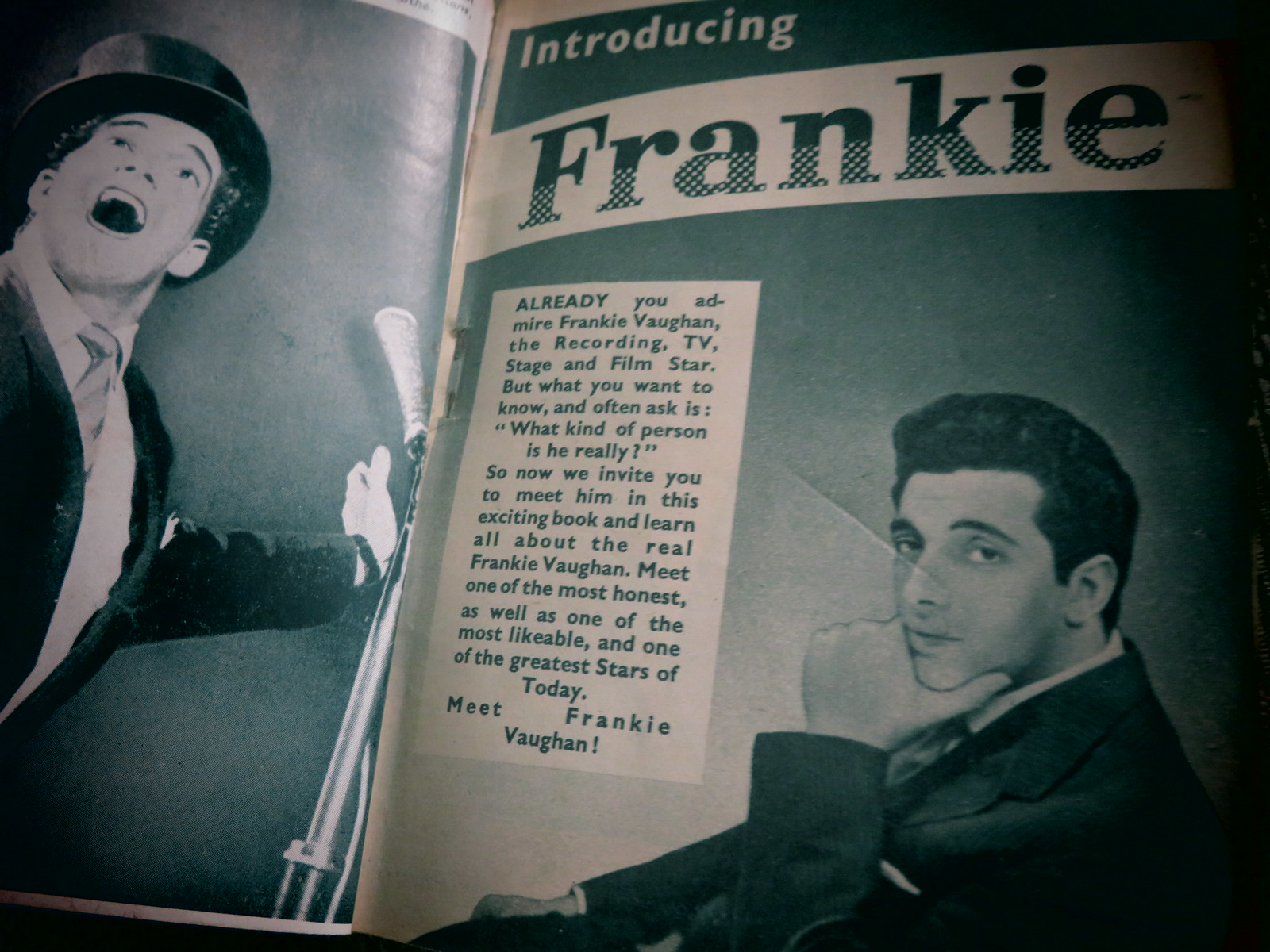This black and white advertisement, possibly from a magazine or periodical, features a striking monochromatic palette that extends to greenish-hued shades of teal. The image spans two pages with a prominent crease in the center. On the left page, there is a performer—Frankie Vaughan—captured in a dramatic pose, wearing a top hat and suit with a microphone poised near his left hand, all set against a dark background. The right page is dedicated to introducing Frankie Vaughan, with bold text reading "Introducing Frankie," followed by a paragraph detailing his multifaceted career as a recording artist, TV, stage, and film star. The text appeals to readers’ curiosity about Vaughan's true personality, inviting them to discover more in an exciting book about "the real Frankie Vaughan." At the bottom right of this page, another image of Frankie Vaughan is depicted: he is seated, dressed in a dark suit that contrasts with his short black hair. His left hand is thoughtfully placed against his chin, giving him a composed, if slightly smug, demeanor. This portrait, with Vaughan looking directly at the camera, underlines his confident yet approachable nature, enhanced by the transitioning white and gray background.